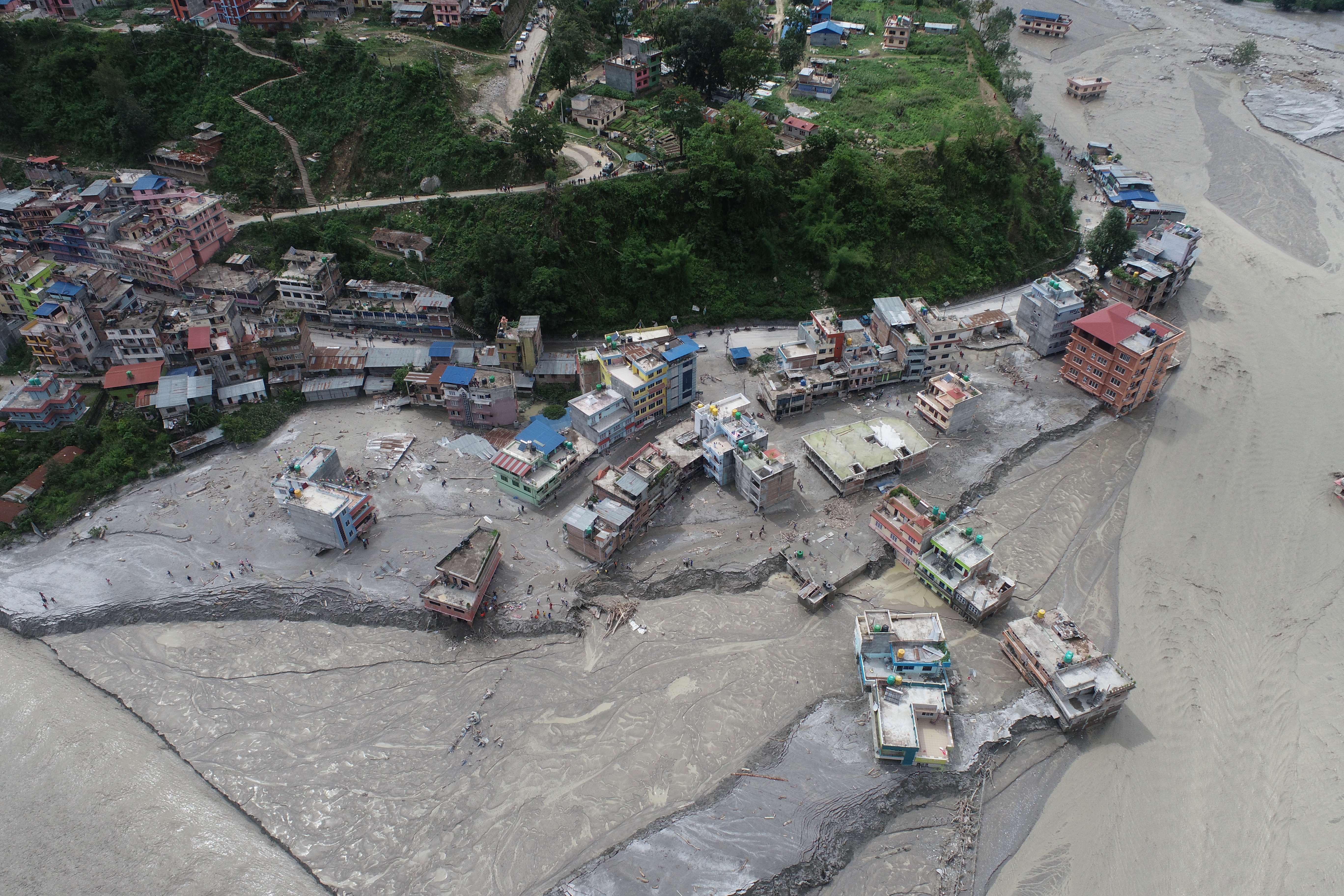This aerial photograph captures a disaster-stricken town that has been severely flooded. The inundated lower region showcases murky, muddy waters that have displaced several buildings from their original positions. The structures, primarily multicolored concrete houses with square windows and balconies, now stand in disarray. The upper region of the town, sitting on a hill, appears to have been spared from the flooding. This elevated area is characterized by a cluster of buildings surrounded by dark green foliage and traversed by a winding road. The overall scene is marked by a dull, gray color palette, with scattered trees and roads cutting through, and small figures visible on sandy patches, hinting at human presence amidst the devastation. The architectural style and building materials suggest that this location is outside the United States.